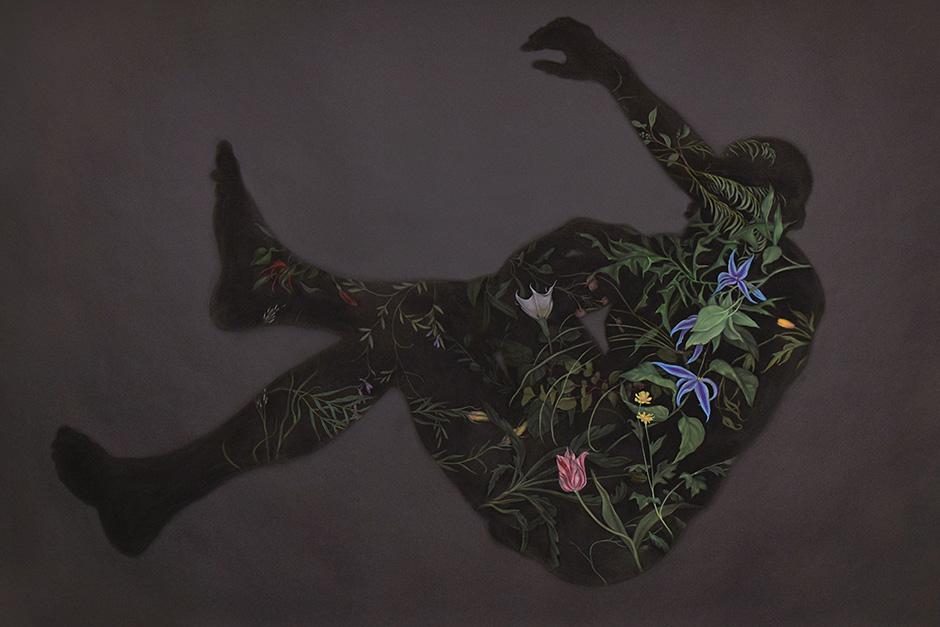This illustration depicts a featureless black silhouette of a man lying on a charcoal gray ground. The man is curled up, almost in a fetal position, with his left arm raised as if shielding his face. The silhouette is richly adorned with an intricate floral pattern, featuring green vines, leaves, and various flowers in hues of red, yellow, blue, and white. These elements are interwoven throughout his entire form, giving a striking contrast against the dark background. The flowers and foliage create a vivid, almost ethereal overlay that embellishes the man's outline, enhancing the abstract nature of the artwork.